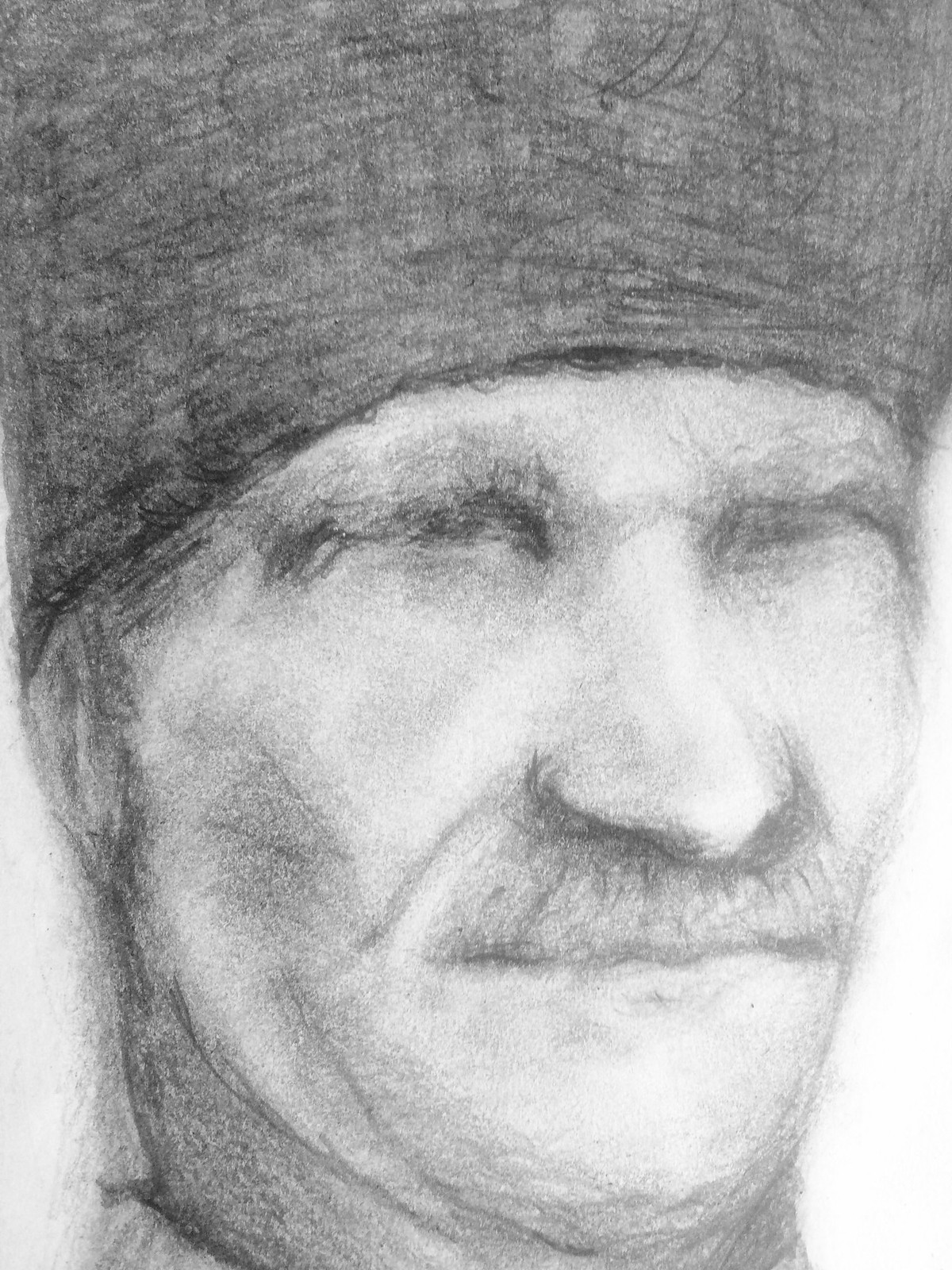A detailed sketch of an older man is presented. He is depicted wearing a black hat that extends beyond the frame, giving an impression of its incomplete visibility. The hat evokes a sense of Russian influence. His facial expression is stern and serious, with one sharply focused eye directed towards the viewer, while the other eye is blurred, adding a sense of mystery. His pointed nose and a small mustache give character to his visage. The artist has skillfully incorporated smile lines at the corners of his mouth and carefully shaded areas to highlight his cheekbones. The neck is deeply shaded to create a realistic shadow, emphasizing the contours of his face and neck. The man's left ear is partially concealed by the hat, further enhancing the enigmatic aura of the portrait.